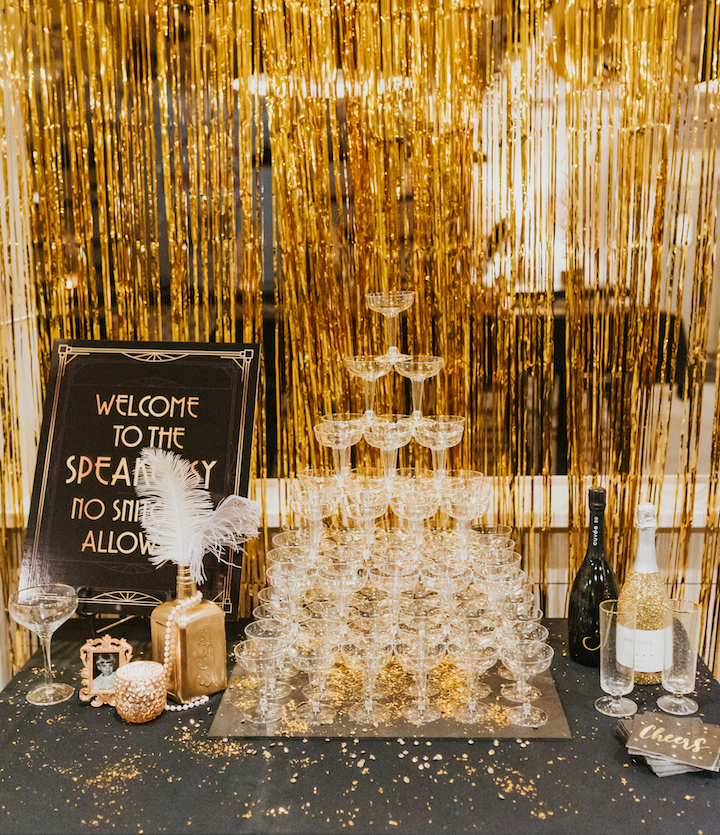This image captures a lavish 1920s-themed celebration, likely a wedding reception or centennial birthday party. At the forefront stands an elegant tower of meticulously stacked champagne glasses, poised for a sparkling toast. The glasses sit on a silver surface adorned with dazzling gold sparkles, reflecting the extravagant atmosphere. To the right, two champagne bottles—one black, one shimmering—stand ready, accompanied by two flute glasses and a pile of black napkins emblazoned with the word "Cheers" in gold.

The backdrop is a cascade of glittering gold streamers, revealing snippets of a chandelier-lit room beyond, hinting at a glamorous setting. On the left, an Art Deco-style sign proclaiming "Welcome to the Speakeasy, No Snitches Allowed" evokes the Prohibition era. Beside it, a liquor bottle adorned with a white feather and a white necklace adds to the vintage charm. A small, ornate gold photo frame displaying a picture of a young child sits nearby, adding a personal touch to the sophisticated display. An air of opulence and celebration permeates the scene, perfectly blending historical nostalgia with festive elegance.